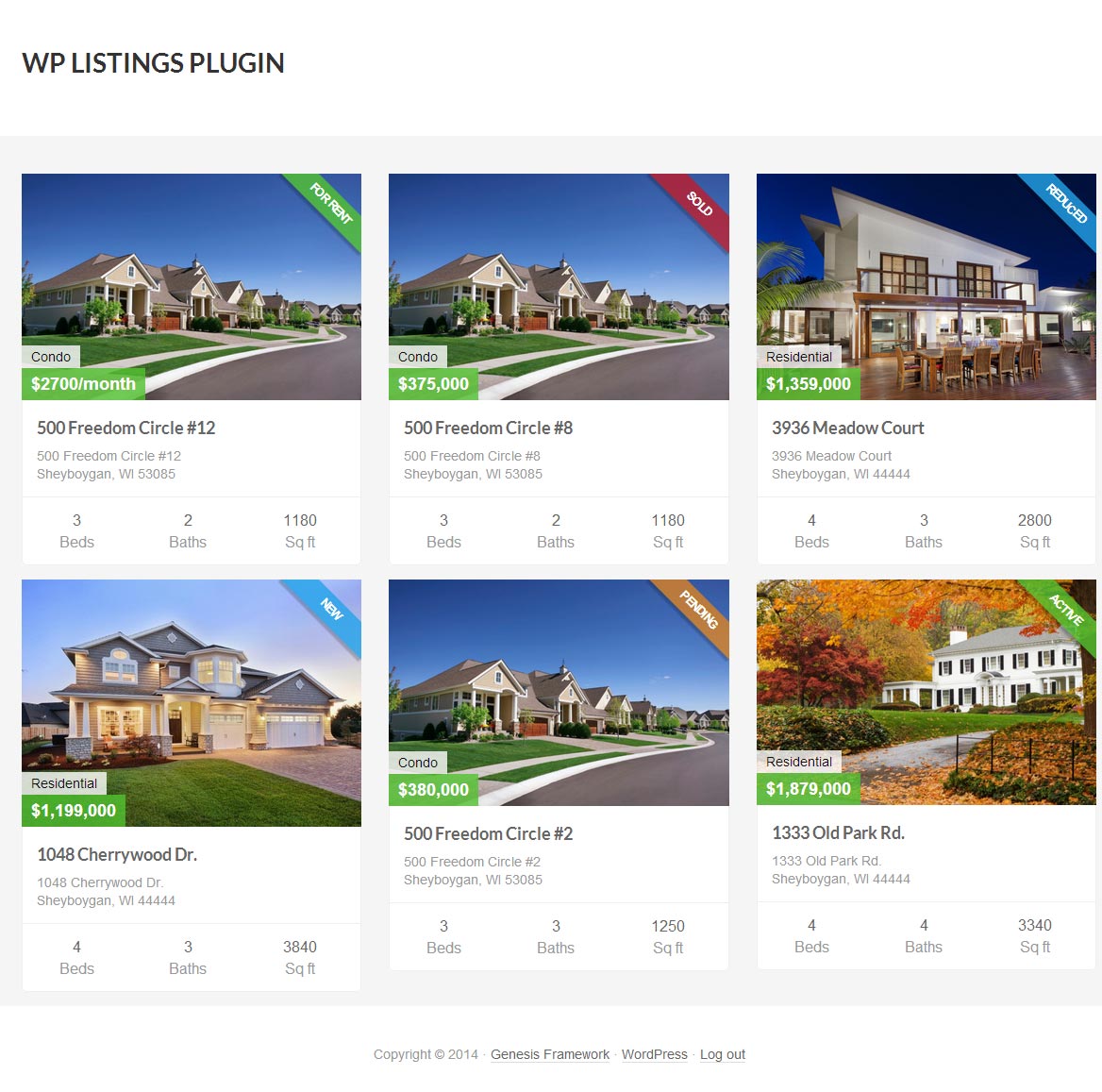A screenshot appears to depict a webpage likely viewed on either a PC or a tablet, showcasing a blend of rental and purchase property listings in Sheboygan, Wisconsin. The layout features six property thumbnails organized in two rows of three images each. In the upper left corner, the header identifies the page as powered by the "WP Listings Plugin," printed in black text against a white background. The properties vary between single houses and identical condos, with detailed information such as prices and addresses displayed beneath each thumbnail. 

Specifically, two of the featured condos on 500 Freedom Circle are listed: one available for rent at $2,700 per month and the other for sale at $375,000. Each listing includes details about the number of rooms and other key features. The overall presentation offers a concise and organized view of available real estate options in Sheboygan.